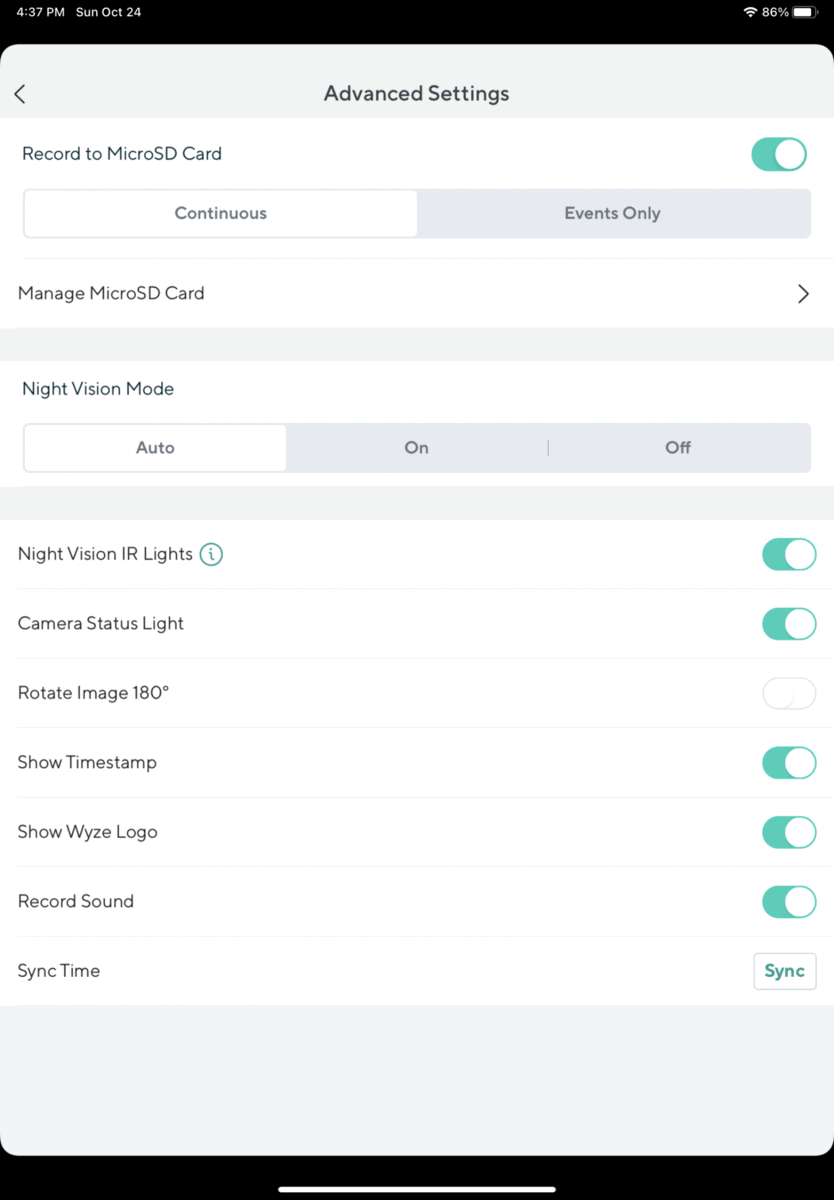The image is a screen capture of a mobile device, either a cell phone or a tablet, displaying a detailed view of an app's advanced settings menu. The information on the screen indicates that it is Sunday, October 24, at 4:37 p.m., with the battery level at 86%.

The settings menu shown includes several configurable options. The recording preference is set to "Record to micro SD card" with the recording mode specified as "Events only." There is an option to manage the micro SD card, represented by a line and an arrow implying it would open another section of the app, though it has not been selected. 

Additional configurable settings are as follows: 
- Night vision mode is set to auto.
- Night vision IR lights are toggled on.
- Camera status light is turned on.
- The option to rotate the image 180 degrees is not enabled.
- The timestamp display is enabled.
- The display of the Wyze (W-Y-Z-E) logo is toggled on.
- Audio recording is enabled with the "Record Sound" option turned on.

At the bottom of the screen, there is a button labeled "Sync" next to the "Sync time" option, indicating the functionality to synchronize the device's time settings when the button is pressed.